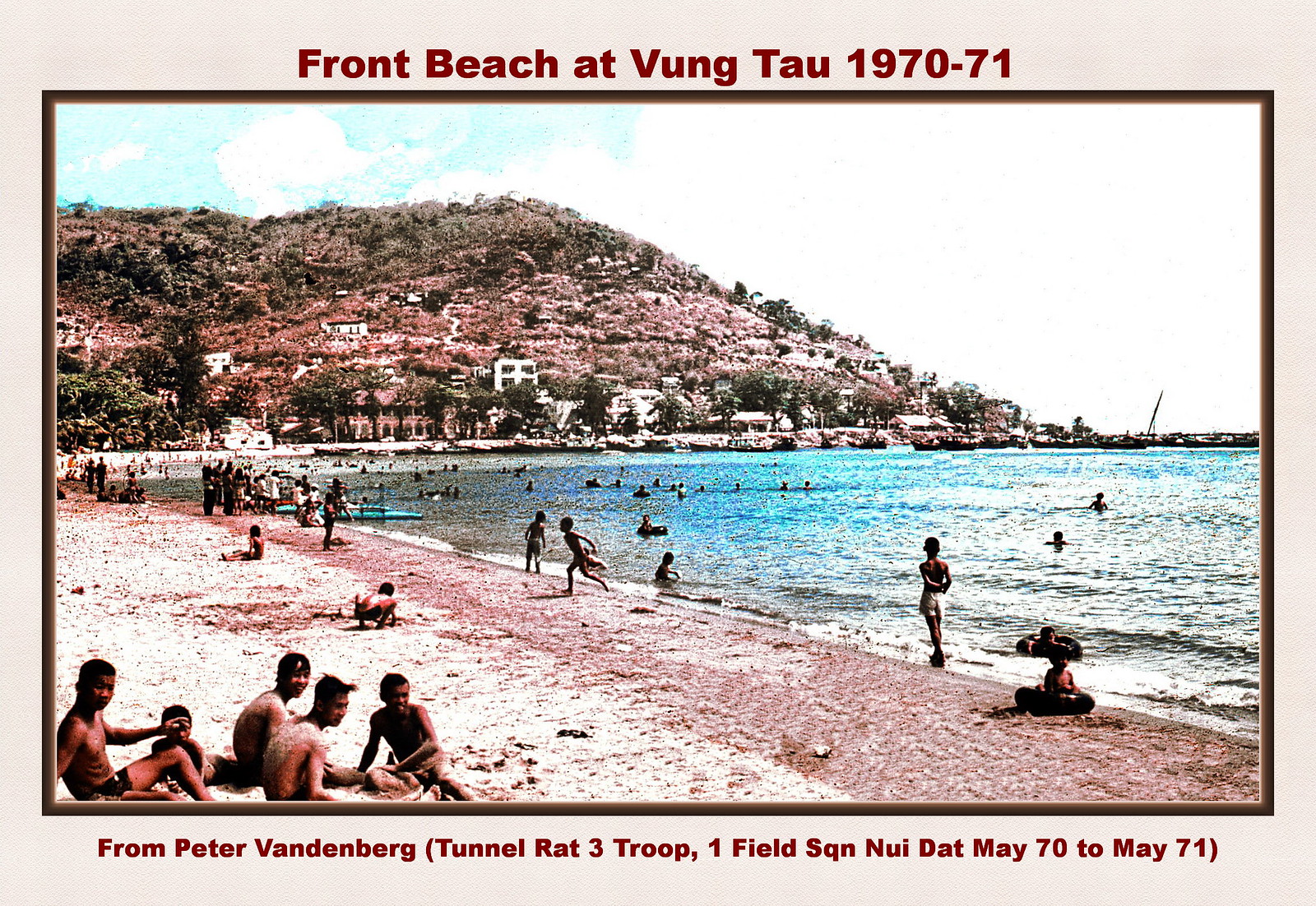This is a horizontally aligned rectangular picture with a light gray border surrounding it. At the top, dark brown text reads "Front Beach at Vung Tau, 1970-71." Below the image, more dark brown text states "From Peter Vandenberg, (Tunnel Rat 3 Troop, Onefields SQN, Nui Dat, May 70 to May 71)." The image itself is bordered in dark brown. The upper left corner of the photo reveals a vibrant blue sky with puffy white clouds, transitioning to a blanket of white clouds occupying the upper right side. 

Central and left areas of the background feature a large hill composed mainly of dirt, rocks, and interspersed trees, with some white buildings and varying shades of brown and green. To the right side, extending to the middle, is a vast area of calm water, fading from blue in the distance to a brownish-gray near the shore. The beach, colored in tones of brown and tan, forms the lower part of the image and hosts an array of beachgoers. Children gather along the shoreline and in the surf, while a group of young men with sand-covered backs can be seen sitting on the beach in the lower left-hand corner. The scene captures a bustling, sunny day at Front Beach during the early '70s.